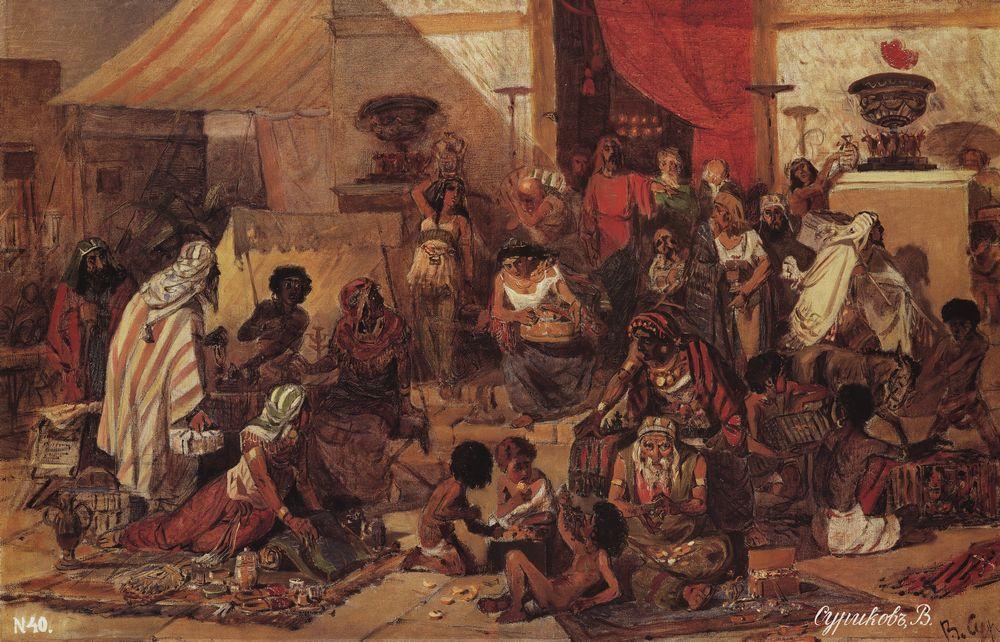This painting by Asen Obkabi depicts a bustling Middle Eastern bazaar, characterized by a rich blend of culture and vibrant activity. The scene is set under a yellow-striped canopy on the upper left, with red tapestries adding a touch of color to the predominantly white-walled backdrop. Spread across the composition are numerous figures adorned in traditional Middle Eastern attire—robes and towel-like headdresses. In the foreground, there are unclothed or barely clothed children playing on the ground, adding a sense of liveliness.

To the left, a woman is seated on a blanket surrounded by various items, while closer to the middle, more children are seated, engaging with each other. An elderly person sits nearby on a blanket facing the viewer. Behind them, a woman appears to be dancing with her arm raised, positioned next to a small tent. The background reveals a large entrance to a building, with its walls partially visible and a large red curtain draped to the side, through which several people are seen exiting. Scattered around the scene are brown vases and other objects, possibly pots or bells, enhancing the historical ambiance of the market. The painting also bears the artist’s signature in the bottom right-hand corner along with the inscription "n40" on the left-hand side.